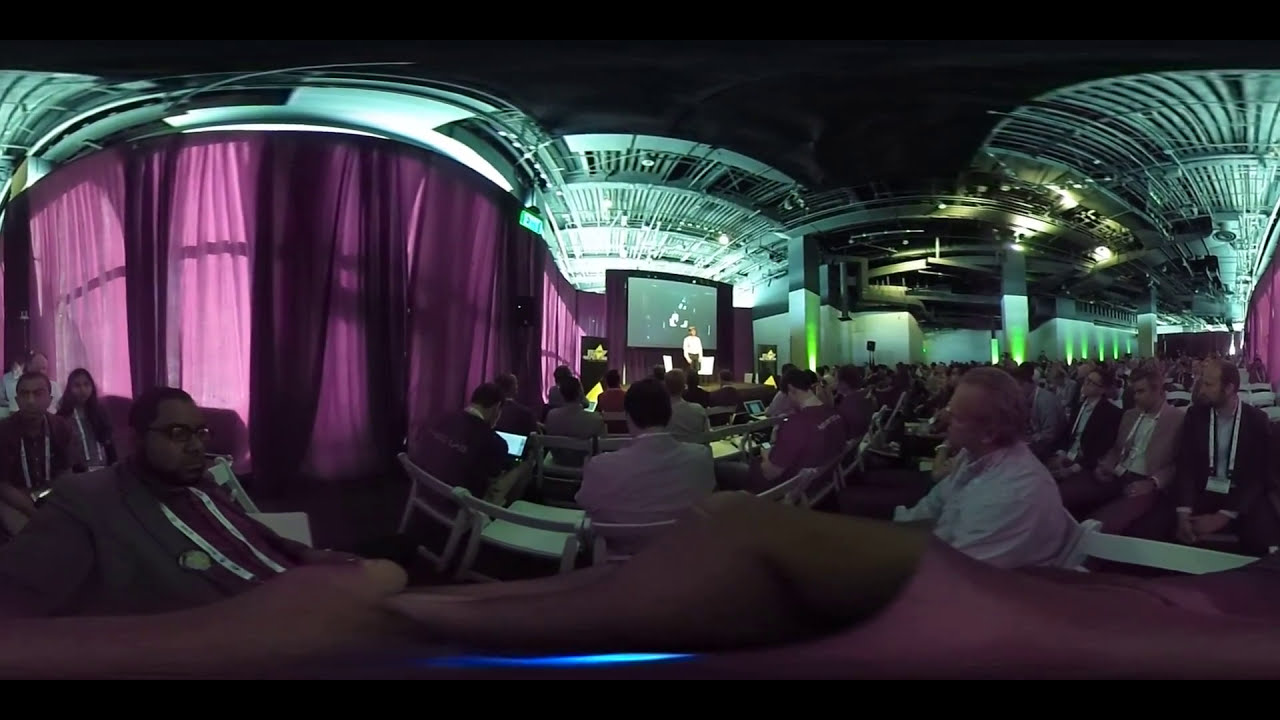The image depicts an expansive conference room, possibly a large ballroom, characterized by a distinct fisheye lens effect that lends a curvature to all elements within the frame. The ceiling is a striking feature, with a black backdrop interspersed with large, scalloped arcs of blue, accentuated by lime green lighting that emanates from the floor. The left side of the image is dominated by vertically hanging purple curtains. In the center back of the room, a speaker dressed in a white shirt and black pants stands on a stage in front of a large projector screen, delivering a presentation. The attendees, identifiable by their lanyards, are seated on white chairs arranged in various orientations — some facing directly towards the stage, while others face inward or appear to be looking straight ahead. The crowd is comprised of people from different backgrounds, some of whom are using laptops. The atmosphere suggests a formal, possibly educational or professional setting, similar to a convention or TED talk. Scattered throughout the room are metal grid frames and pillars, and in the foreground, the image inadvertently captures a thumb at the bottom edge, further emphasizing the fisheye distortion that gives the image its unique bubble-like effect.